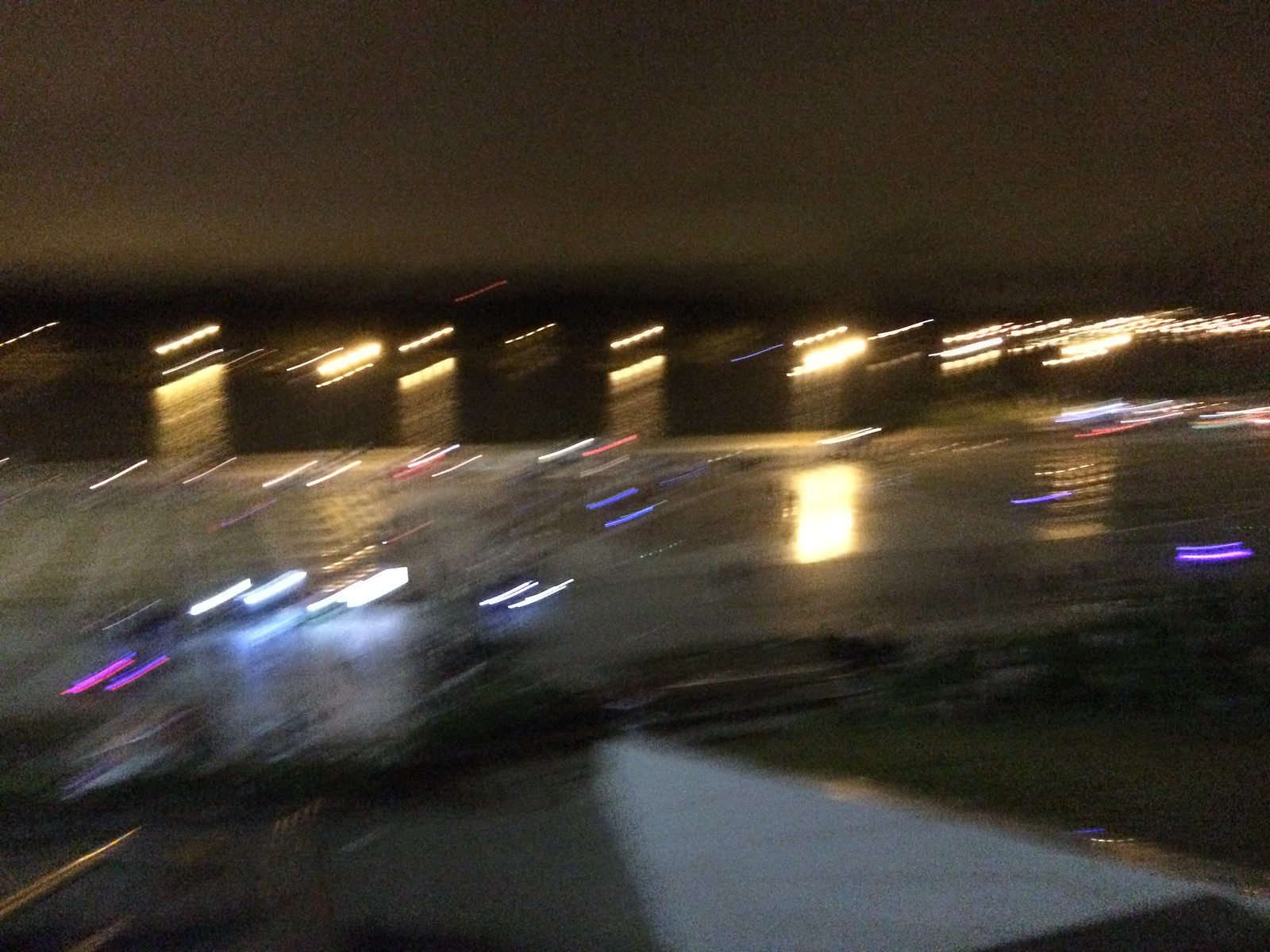The image captures a highly blurred aerial view of an urban landscape at night. On the left side of the image, there is a ground area shaded in gray, featuring a couple of indistinct, rod-like objects tinged with gold. The center bottom section showcases a light gray strip, transitioning into a green area to its right. Slightly to the left of this green section, there appear to be a few building structures adorned with light fixtures; the lights form distinct rectangular, diagonal patterns in shades of white and light blue, alongside a touch of pink light on the lower left side of one of the buildings.

Across the rest of the image, a series of slender, diagonal lights in white, red, and blue can be seen, adding a dynamic feel to the scene. In the distant background, yellow lights from buildings create a blurred, hazy effect. The top portion of the image is dominated by a sky appearing in an intensely dark brown hue, adding to the nighttime ambiance of the photo.